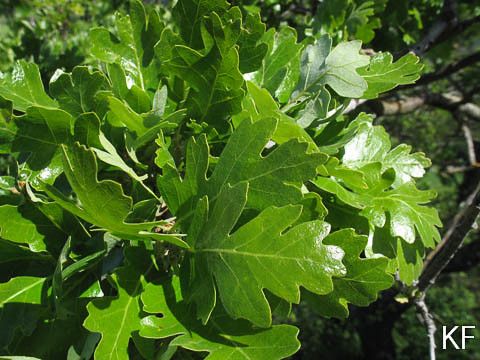This detailed image captures a close-up of a vibrant clump of green leaves, most likely from a type of tree, possibly resembling oak leaves. These leaves are large, thick, and have a detailed, textured surface with ridges and multiple points. Their fresh and healthy appearance suggests the photo was taken during spring or summer. The leaves appear bright green, with lighter green veins, and sunlight reflecting off their surface enhances their shiny, vibrant look. In the background, there are thin, dark grayish branches weaving in and out, adding depth to the scene. The focus is primarily on these clustered leaves, which stand out against the minimal brown elements. In the lower right corner of the image, the initials "KF" are subtly visible in white, possibly indicating the photographer's signature. The overall composition highlights the lush, green vitality of nature.